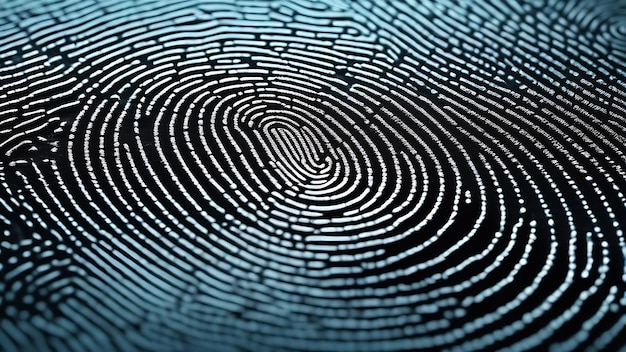The image is a highly abstract and close-up rendering that evokes the intricate patterns of a fingerprint. The background is predominantly black, with swirling lines creating a striking contrast in shades of blue and white. These lines form a series of concentric swirls that start tightly packed and detailed at the center, where the fingerprint-like pattern is most apparent. As the lines radiate outward, they become more spaced out, blurred, and less regular, blending more into blue tones and creating a sense of motion and fluidity. The image is characterized by both long, continuous lines and shorter, broken ones, producing an irregular, almost chaotic pattern that lacks a discernible repetition. The middle of the image is dominated by the black background, while the edges are more saturated with the blue and white swirls, enhancing the overall abstract and dynamic quality of the piece.